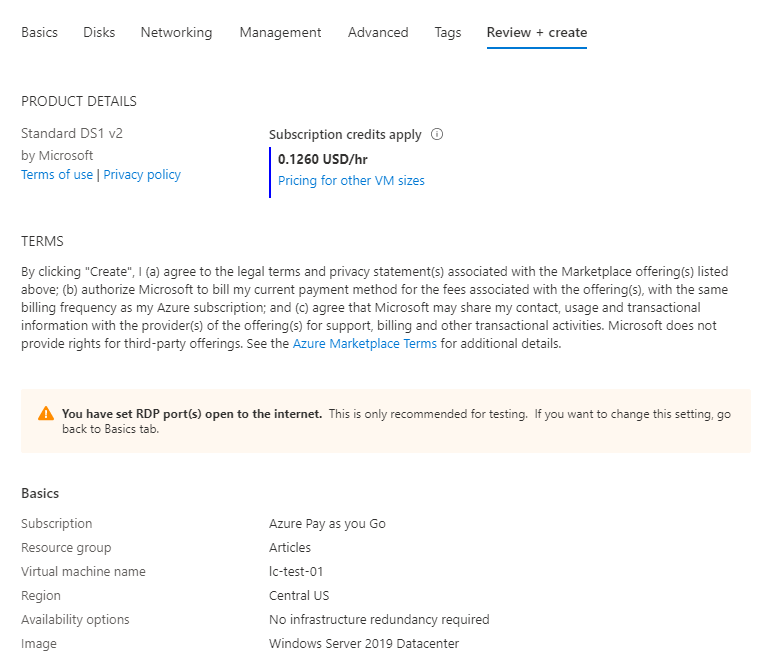The image is a screenshot of a cloud service configuration page, primarily displaying on a white background with specific sections detailed for setup. 

In the upper left-hand corner, there are tabs labeled "Basics," "Disks," "Networking," "Management," "Advanced," and "Tags," with the "Review + Create" tab highlighted with a blue line underneath and in bold text, indicating the current page.

The next row contains details specific to the product: "Product Details," showing "Standard DS1 by Microsoft." Below this, in light blue text, are the live links "Terms of Use" and "Privacy Policy." A purple line beneath these links states "Subscription Credits Apply, $0.1260 USD per hour," and another live link in light blue text reads "Pricing for Other VM Sizes."

A note in italics states, "By clicking Create, I agree to the legal terms," followed by a section in blue with a live link labeled "Azure Marketplace Terms."

An overlay section with a tan background and an orange exclamation point triangle contains a warning: "You have set RDP ports open to the internet. This is only recommended for testing. If you want to change the setting, go back to the Basics tab."

The page layout then shifts into two columns: 
- The left column under "Basics" includes:
  - "Subscription" with the entry "Pay-As-You-Go"
  - "Resource Group" with the name "Articles"
  - "Virtual Machine Name" (not detailed in the description)

- The right column covers further details:
  - "Region" set to "Central US"
  - "Availability Options" showing "No Infrastructure Redundancy Required"
  - "Image" displaying "Windows Server 2019 Datacenter"

This screenshot provides a detailed view of the setup and pricing information for creating a virtual machine on Microsoft's Azure platform, along with important warnings and terms of use.